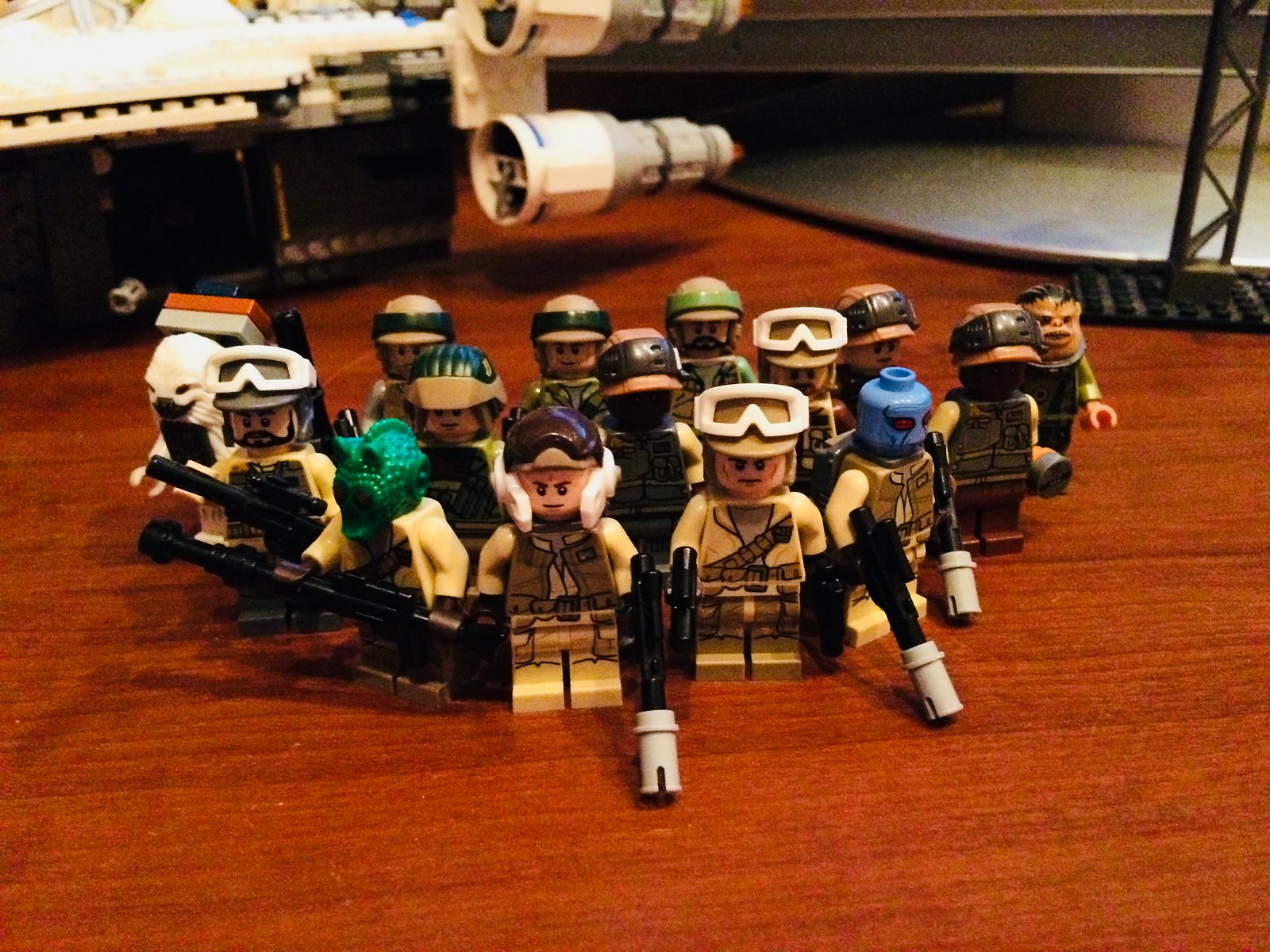In the image, a group of approximately 20 Star Wars licensed Lego figurines is arranged in a triangular formation, similar to the setup in pool. These blocky figurines feature various connecting points typical of Lego toys and are standing on what appears to be a wooden desk or table. They wear matching khaki uniforms, complemented by brown vests, bandoliers, and sport little plastic guns with silver tips. Some figurines are equipped with additional accessories like goggles, helmets, and visors, while others resemble alien creatures or fighter pilots. In the background, a detailed Lego spaceship with four engines and a cockpit is visible, accompanied by a computer monitor in the top right corner. The setting is an indoor space, possibly a child's room, filled with rich colors including brown, black, white, yellow, green, and blue.